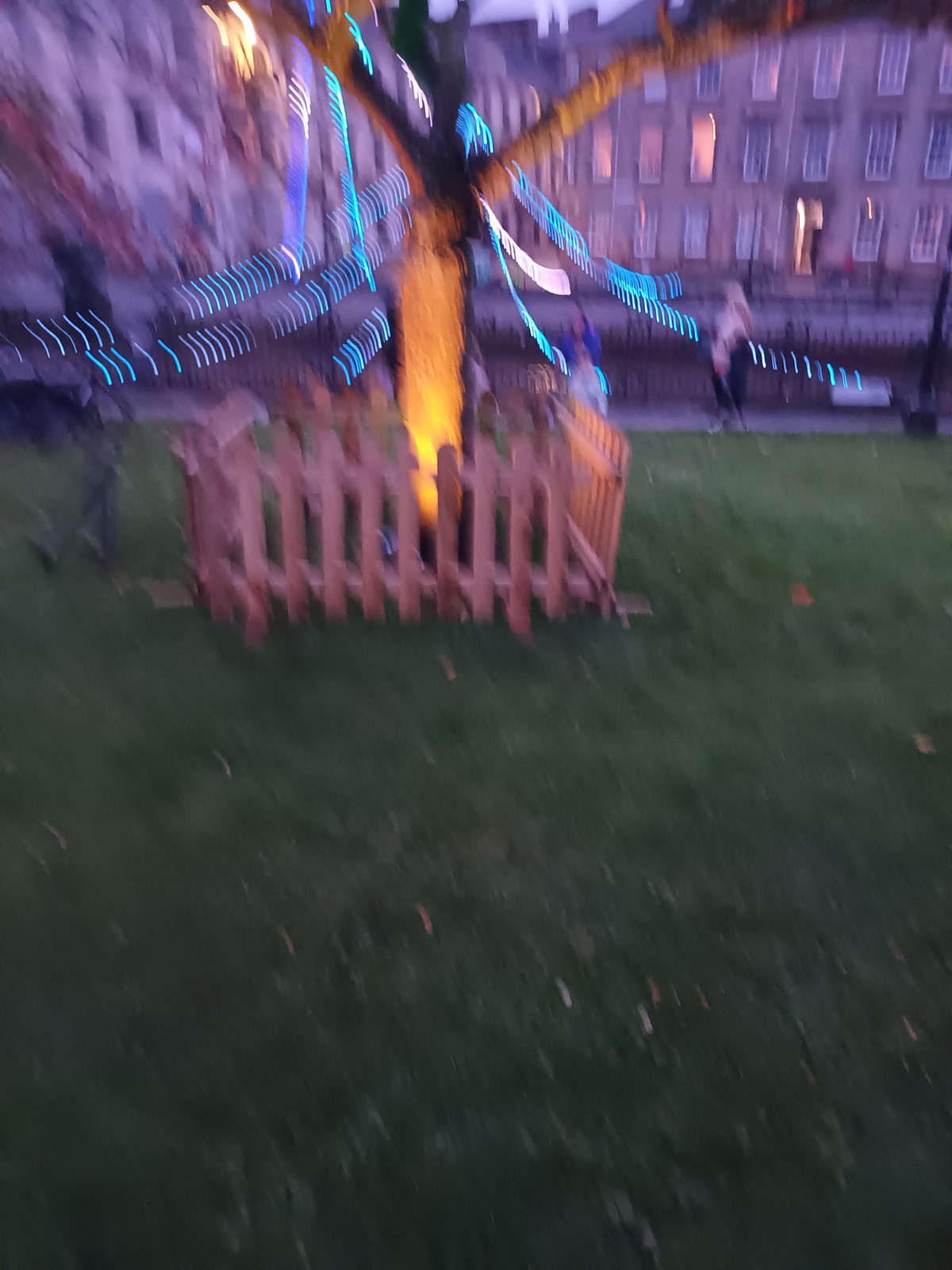This is a blurry photograph taken outside, possibly in the early morning or at nightfall, capturing what seems to be a backyard scene. Central to the image is the lower portion of a tree, illuminated by a light at its base. The tree is encircled by a light brown, square wooden picket fence. Emanating from the tree are strands of fuzzy, blue-purple lights. The tree is situated on a large, flat grassy area. In the background, there stands a long, white apartment building with many rectangular windows, some of which are lit up, especially on the right side. A sidewalk runs in front of this building, and there are faint, blurry images of people scattered around the scene.